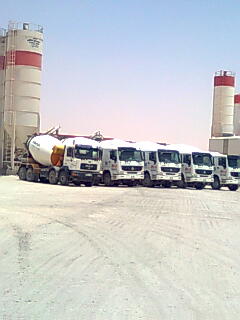This image depicts an industrial lot featuring a line of five concrete mixer trucks parked diagonally and facing the camera. Each truck has a white cab and is equipped with a cylindrical mixer drum at the rear, used for mixing and transporting concrete. The drums are primarily silver and appear to be part of a cohesive fleet belonging to the same company. The trucks are positioned on an unpaved, sandy, and dusty ground, common in construction and industrial areas, with visible tire tracks suggesting regular activity. In the background, tall cylindrical silos are prominently displayed; these white silos with red bands near the top are used for storing bulk materials like cement. One of the silos has an attached ladder leading to a fenced platform at the top, indicating it is designed for maintenance and operational access. The sky above is clear, transitioning from blue at the top to a subtle pink near the horizon, suggesting a sunny day. The composition of the image, with the trucks in the foreground and silos in the background, effectively conveys a bustling industrial setting.